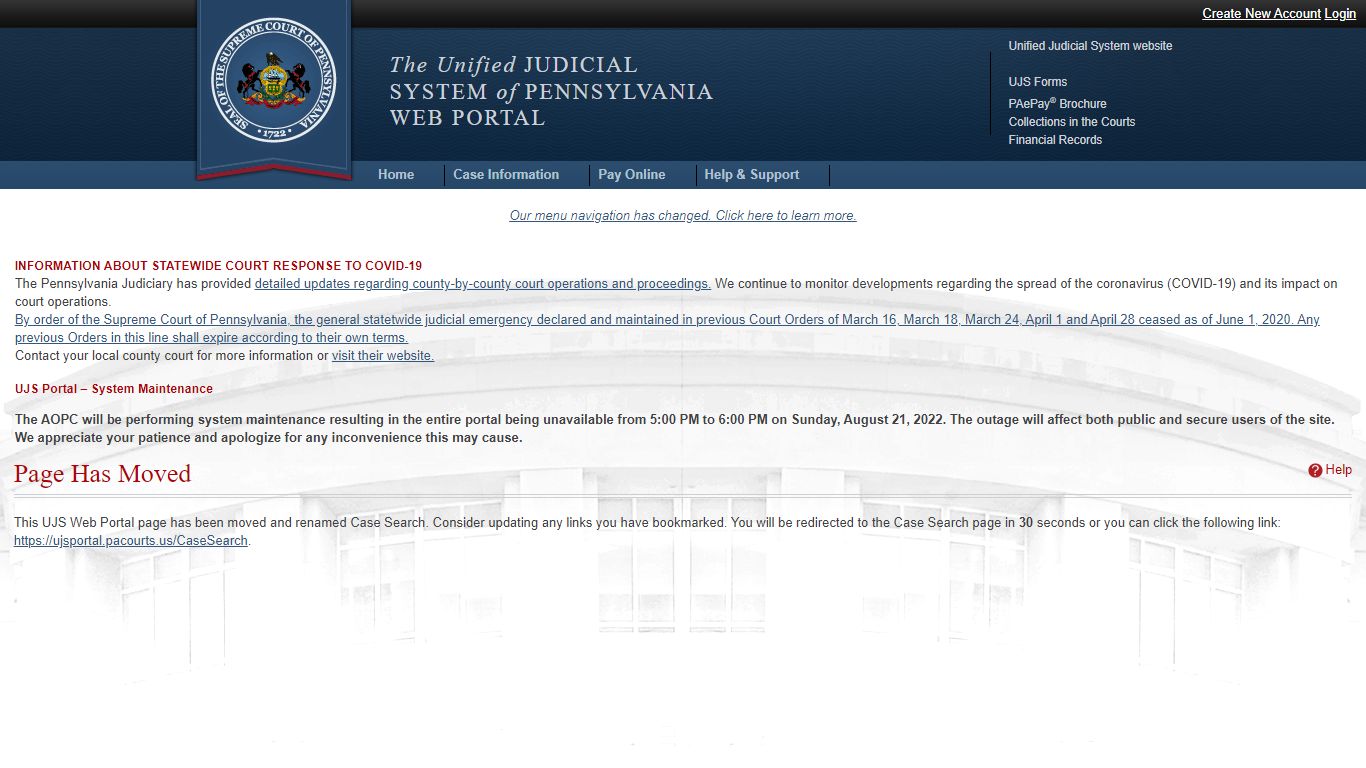The image features the web portal homepage for the Unified Justice System of Pennsylvania. The background at the top is a gradient of grayish black. Positioned slightly to the right of the left-hand side is the state seal of Pennsylvania, embellished with black horses and some sort of crest. Although encircled by text, the exact words are indecipherable. Adjacent to the seal, white text reads "The Unified Justice System of Pennsylvania Web Portal." 

On the right-hand side, there is additional white text above a black bar, but its content is unclear. Within the black bar, an underlined white text appears to say "Create New Account / Log In." Below this, a lighter blue section contains the website's main navigation tabs labeled 'Home,' 'Case Information,' 'Pay Online,' and 'Help and Support' in white text.

The page continues with a profusion of black and very light gray text, unreadable due to the small font size. Notably, on the bottom left, a prominent bullet point reads "Page has moved." On the bottom right, only the word "Help" is partially legible, followed by more unreadable white and gray text.